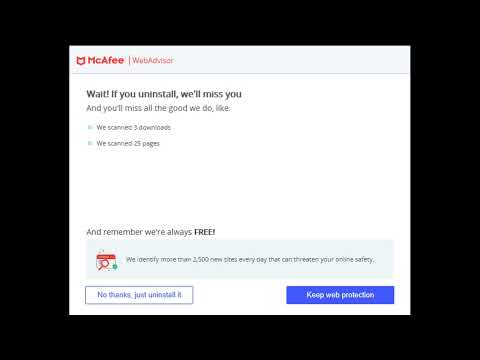The image features a black rectangular background with a white (or light gray) rectangle inside it. In the upper left corner of the white rectangle, the word "McPhee" is written next to a logo. Below this, a line of text reads: "Wait! If you uninstall, we'll miss you, and you'll miss all the good we do." There is a light gray dot followed by the word "Welcome" and another light gray dot with more text that is not legible.

Further down, a line states: "And remember, we're always free!" Below this, there is a light blue rectangle and an image of a red outlined rectangle with a red bar across the top, accompanied by a magnifying glass icon. The text next to this image is too small to decipher.

Finally, at the bottom of the white rectangle, there are two buttons. The first is an outlined rectangle with blue text that reads: "No thanks, just uninstall." The second button is filled with blue and partially reads "Keep with," but the rest of the text is unclear.